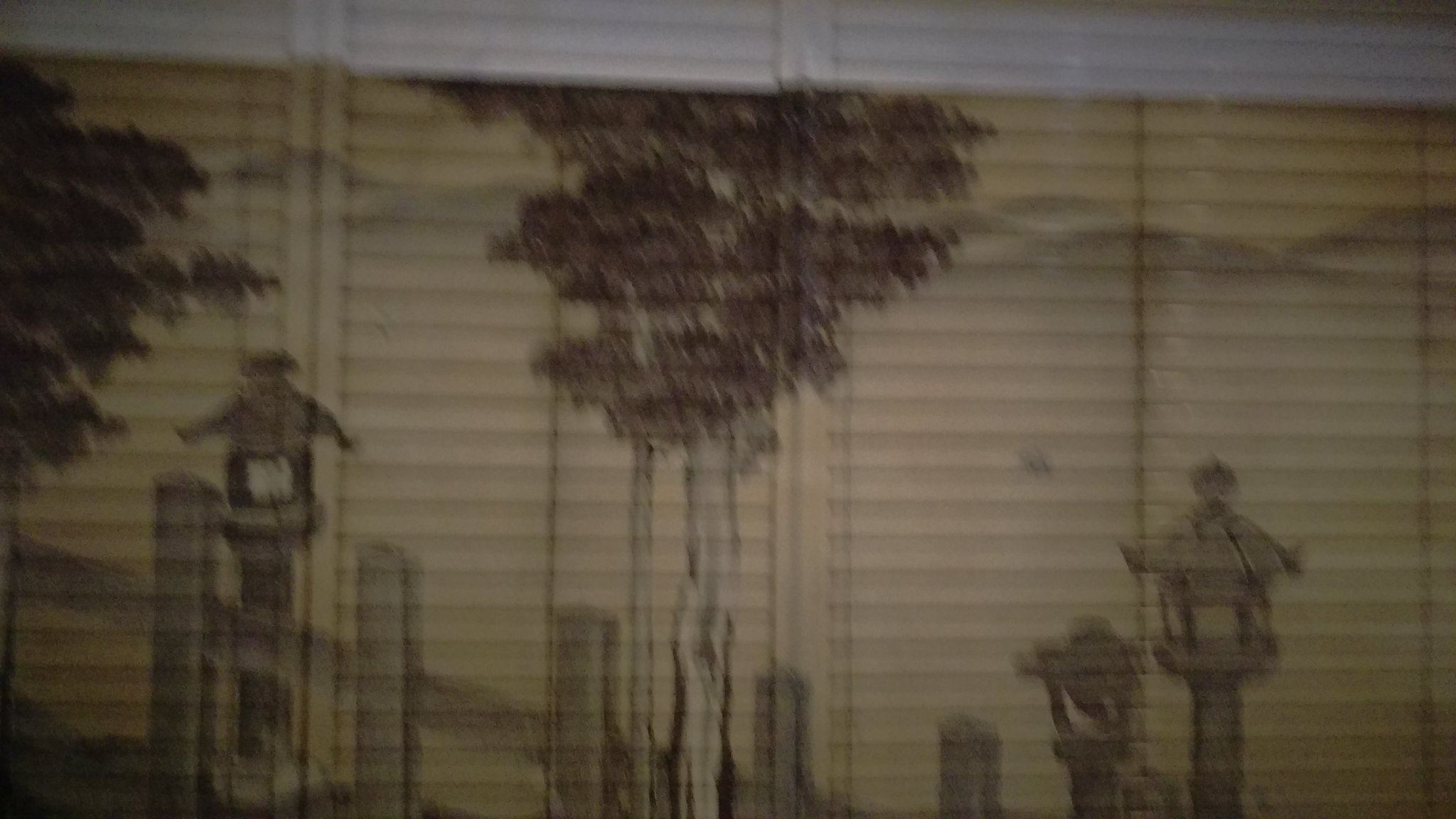A grainy, dimly lit exterior night photo captures the horizontally rectangular side of a building in a blurry fashion. The building’s siding consists of horizontal wooden slats. At the very top of the frame, the wall is white, but it transitions into a dark beige-ish yellow for the remainder of its height. A mural adorns the wall, featuring a tree that rises from the bottom center and spreads its branches and leaves upwards. Towards the top of the image, a simple picket fence extends from the bottom center, diagonally upwards to the left. Behind the fence, there are two totem-like figures, though their details are too obscure to discern clearly. The mural incorporates dark colors, possibly blacks or reds, and appears to have an Asian-inspired influence, with elements resembling rotund figures in traditional attire standing among the trees. The overall photo is dingy and unclear, making it difficult to make out specific colors and finer details.